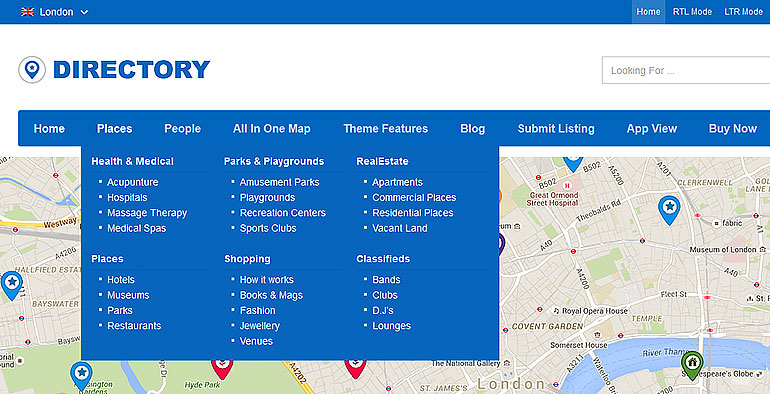This image appears to be a user interface mockup from a computer application. The layout is very structured, featuring multiple colored bars and menus. 

At the very top, there's a narrow instakill bar. Below this, there is a wider white bar, and then a blue bar, followed by a detailed map.

The topmost blue bar displays, on the left-hand side, an English flag beside the word "London" with a drop-down arrow. On the right side of this bar, there are options in white text: "HOME," "RTL MODE," and "LTR MODE." 

Beneath this blue bar, the white bar contains the word "DIRECTORY" in uppercase blue letters on the left. At the far right end of this bar, there is a search bar with the placeholder text "Looking for" in gray.

Further down, there is a second blue bar, which features several menu options in white text: "HOME," "PLACES," "PEOPLE," "ALL IN ONE MAP," "THEME FEATURES," "BLOG," "SUBMIT LISTING," "APP VIEW," and "BUY NOW."

Directly below this bar, there is a categorized drop-down menu structured as follows:

- **Health and Medical**
  - Acupuncture
  - Hospitals
  - Massage Therapy
  - Medical Spas
- **Places**
  - Hotels
  - Museums
  - Parks
  - Restaurants

Next to "Health and Medical," another category labeled **Parks and Playgrounds** includes:
  - Amusement Parks
  - Playgrounds
  - Recreation Centers
  - Sports Clubs

To the right of "Parks and Playgrounds," there is a **Shopping** category consisting of:
  - How It Works
  - Books and Mags
  - Fashion
  - Jewelry
  - Venues

Adjacent to "Shopping," the **Real Estate** category lists:
  - Apartments
  - Commercial Places
  - Residential Places
  - Vacant Land

Finally, the **Classifieds** section includes:
  - Bands
  - Clubs
  - DJs
  - Lounges

The image showcases a comprehensive and organized user interface design, focused on various categories for easy navigation.